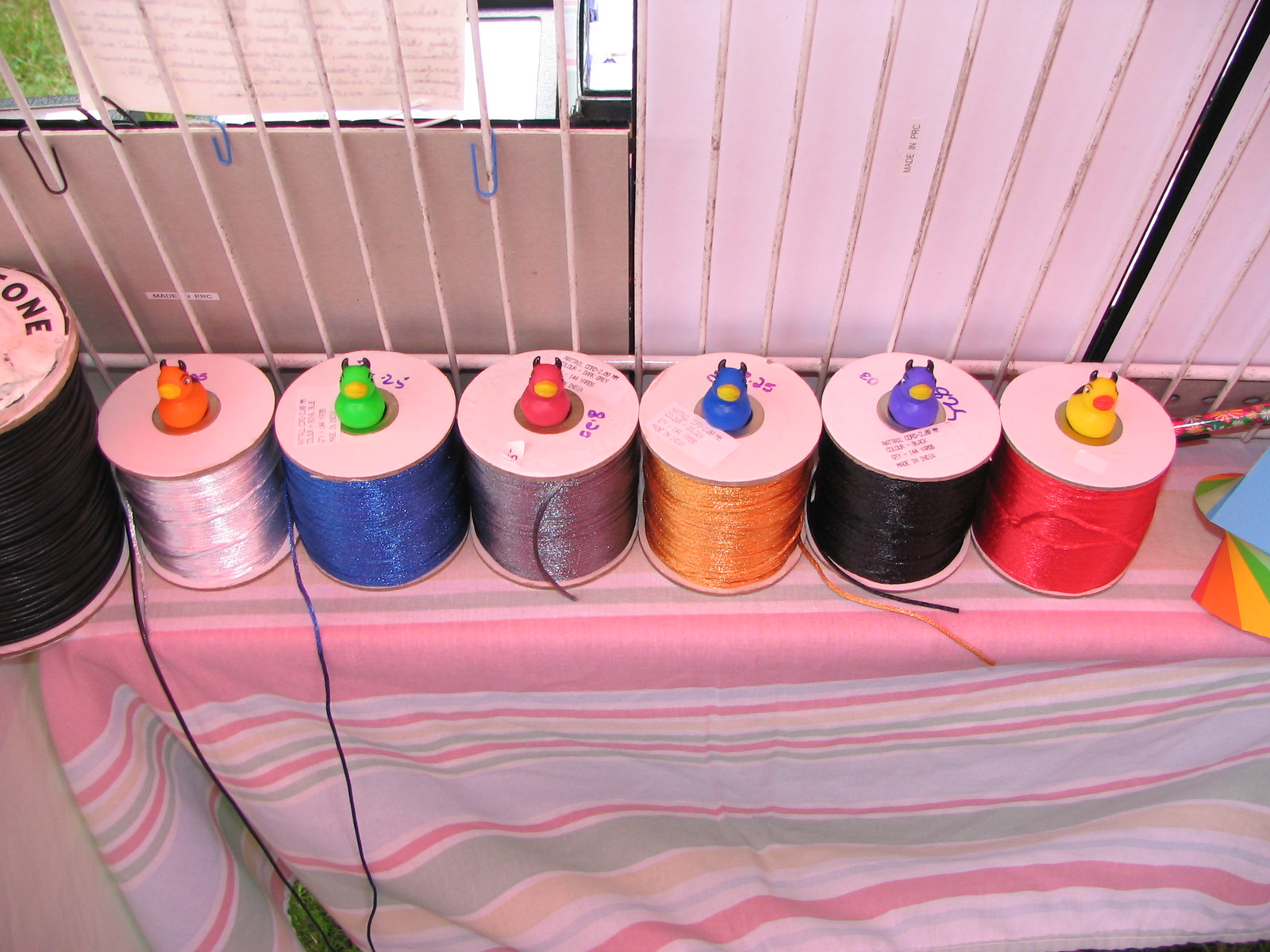The photo depicts a collection of spools of colorful thread arranged in a row on a narrow shelf draped with a large, pastel-striped blanket that resembles a baby blanket. Each spool supports a unique small rubber duck figurine, all adorned with horns resembling those of bulls. The assortment includes ducks in various colors: orange, green, pink, blue, purple, and yellow. The threads themselves are equally vibrant and diverse: white, sparkly light blue, purple, orange, black, coral, gray-silver, orangey-gold, and pink. An additional larger spool, partially visible, edges into the top left corner of the image, introducing another element of black thread. The scene is set indoors, with hints of additional arts and crafts materials and a window in the background, allowing daylight to cast a soft illumination over the array.